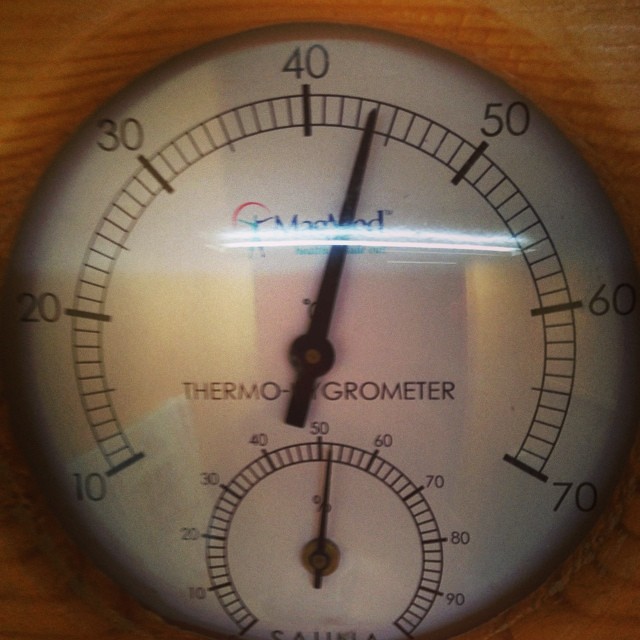The image is a highly detailed, extreme close-up, photorealistic photograph of a circular thermometer that occupies most of the frame. The primary thermometer is centered and features a loop of numerical notches starting at 10 in the bottom left and ascending incrementally through 20, 30, 40, 50, and 60, before descending to 70. Between each main notch are smaller black lines indicating individual degrees. 

In the lower central region of the thermometer is a smaller, nested loop with its own measuring needle, spanning from 0 to 100 in increments of 10. Beneath this smaller dial, partially obscured text appears to spell out "SAUNA". The edges of the thermometer showcase a wooden grain, suggesting it is set into a wooden panel.

At the center of the primary dial, there is an illegible logo due to the reflection of light. However, the text "THERMOGROMETER" is visible beneath the main needle. Additionally, faint reflections in the glass surface hint at a sauna room with yellow walls and a central black entryway.